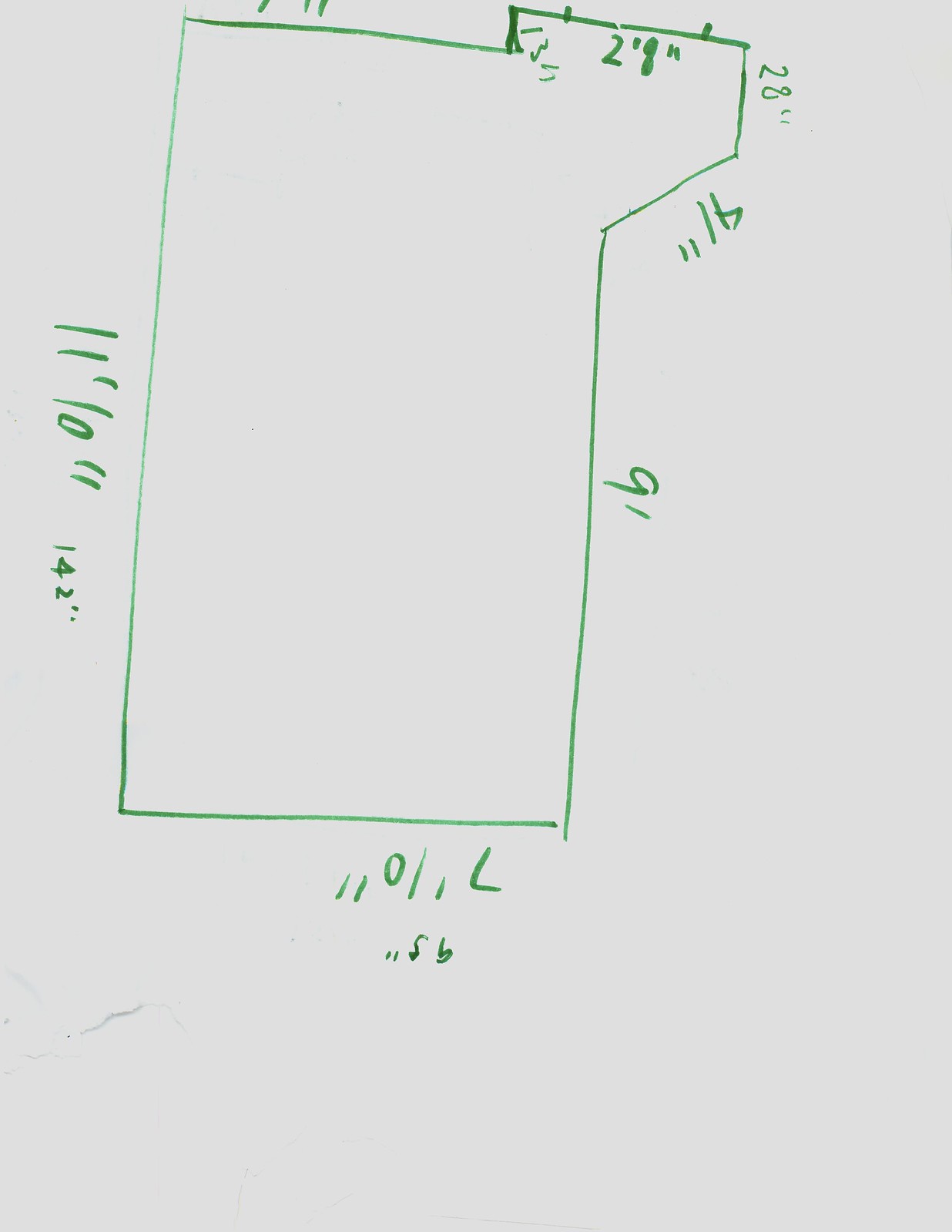This detailed caption describes an image of a hand-drawn diagram on plain white paper, created using a green marker. The main figure in the drawing is a rectangle that slightly deviates at the upper right corner, forming an extension from what appears to be a triangle. This deviation adds an interesting architectural feature to the otherwise straightforward rectangular shape.

Around the perimeter of the drawing, specific measurements are annotated, providing detailed dimensions of various sections. Along the right side of the rectangle, the measurement reads "9 feet," while the bottom edge is marked with "7 feet 10 inches," and positioned below that is the number "56." On the left side, the length is noted as "11 feet 0 inches," with the subsequent number "142." The top of the diagram features the notation "2 feet 9 inches," and the right side additionally shows "28 inches." Another key measurement, "41 inches," is also present, though the exact location is less distinctly mentioned.

This drawing, possibly a room diagram, seems to outline the dimensions and possible expansions of a rectangular space, illustrating an area with great attention to detail through its specific measurements and slight geometrical deviation at the upper right corner.